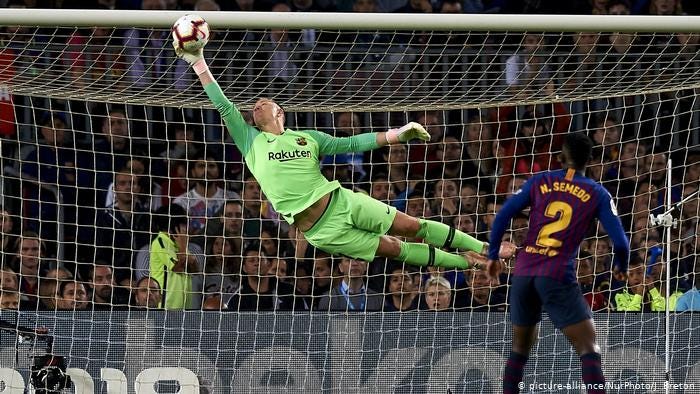In this captivating photograph taken during an intense soccer match, a goalie clad in a green Rakuten long-sleeved jersey, matching green shorts, and tall green shin guard socks, leaps with impressive agility to block a white soccer ball with black and red markings. The goalie, displaying remarkable focus and anticipation, extends his hand high in front of the net, just moments away from deflecting the shot. His dark skin and determined expression highlight his commitment to preventing the goal. Spectators behind the net appear mesmerized by the dramatic scene unfolding before them. On the right-hand side of the image stands an opposing player, his face reflecting surprise and frustration. He is wearing a striking purple jersey with blue sleeves and shoulder, with the text "N. Cimetto" and the number two in yellow on the back, and blue shorts. In the bottom right-hand corner of the photograph is a white-text copyright notice reading, "Picture Alliance, NER Photo, Jay Breton," marking this thrilling moment as a testament to the goalie's athletic prowess during the high-energy game.